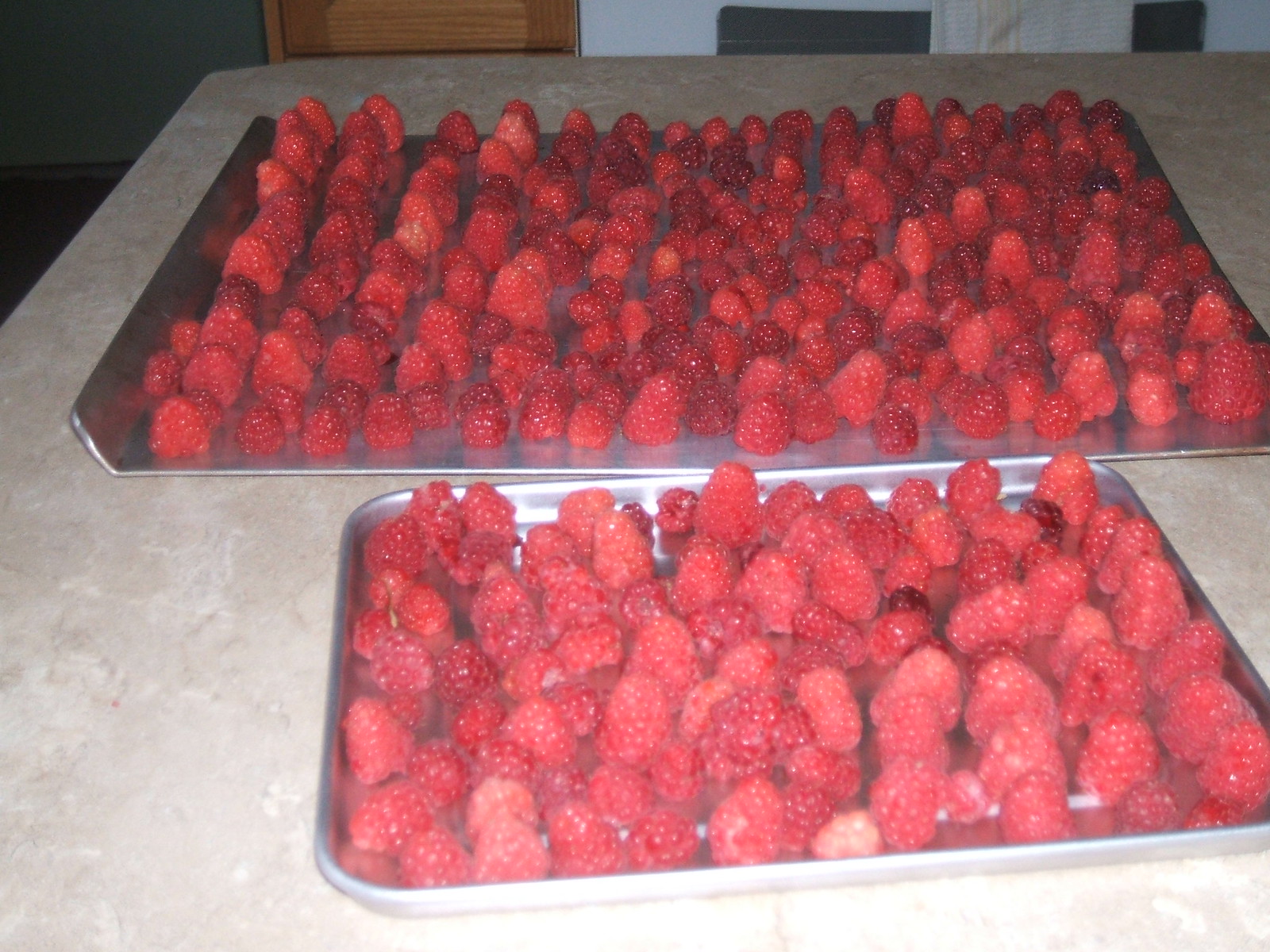In the image, there are two silver baking sheets filled with around 200 fresh raspberries, each meticulously laid out in single layers without overlapping, positioned upright with their holes facing down. The raspberries vary in size and display a spectrum of red hues, signifying different levels of ripeness. These trays rest on a stone-like countertop that appears to be either quartz or granite in a kitchen setting. Behind the trays, a wooden cupboard and possibly a range oven are partially visible, providing context to the kitchen environment.